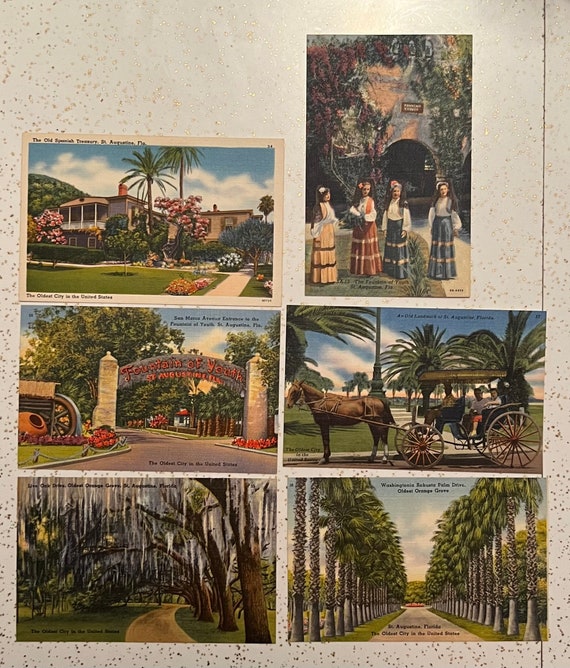This image showcases an arrangement of six old and possibly vintage postcards, displayed against a white marble background, possibly a wall or countertop. The top left postcard features a quaint house surrounded by a meticulously kept lawn and vibrant, colorful trees, including palm trees and flowering trees. Next to it, the top right postcard depicts four girls in traditional dresses standing in front of what appears to be an old building. 

In the second row, the left postcard displays a sign that reads "Fountain of Youth," with a road running beneath it and trees in the backdrop. To its right, another postcard shows a horse-drawn carriage carrying two passengers, with tropical trees gracing the grassy field behind them.

The bottom row begins with a postcard of a willow tree, its white leaves hanging over a dirt path that stretches into the distance. The final postcard on the bottom right illustrates a pathway bordered by tall tropical trees. Despite the presence of captions on these postcards, the text is too tiny to be legible.